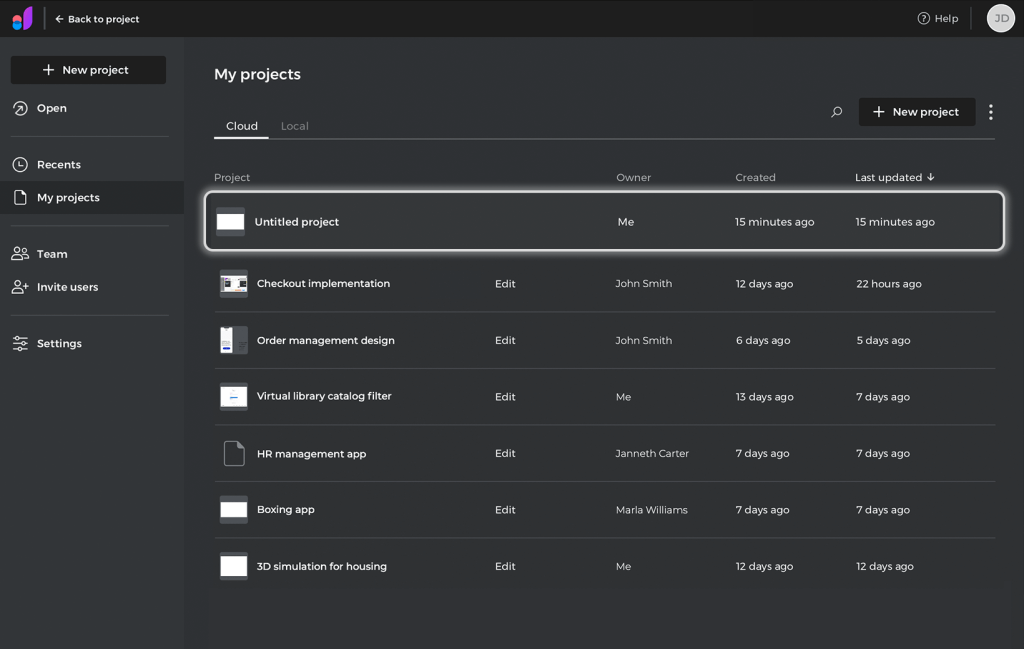**Website Interface Description:**

The website features a dark-themed background, predominantly black or grayish-black. At the top center of the page, a heading labeled "My Projects" stands prominent. Just below the heading, two tabs labeled "Cloud" and "Local" are present, with the "Cloud" tab being highlighted.

On the top right corner, there's a sleek black button labeled "+ New Project" accompanied by a small magnifying glass icon, hinting at a search function.

Below the "Cloud" and "Local" tabs, a well-structured table organizes project details. The table columns are titled "Project," "Owner," "Created," and "Last Updated." Each row in the table lists a project, with details as follows:

1. **Untitled Project**
   - Owner: Me
   - Created: 15 minutes ago
   - Last Updated: 15 minutes ago

2. **Checkout Implementation**
   - Owner: Varies
   - Created: Various times
   - Last Updated: Different times

3. **Order Management Design**
   - Owner: Varies
   - Created: Various times
   - Last Updated: Different times

4. **Virtual Library Catalog Filter**
   - Owner: Varies
   - Created: Various times
   - Last Updated: Different times

5. **HR Management App**
   - Owner: Varies
   - Created: Various times
   - Last Updated: Different times

6. **Boxing App**
   - Owner: Varies
   - Created: Various times
   - Last Updated: Different times

7. **3D Simulation for Housing**
   - Owner: Varies
   - Created: Various times
   - Last Updated: Different times

On the far left of the screen, a slim vertical sidebar provides additional navigation options. At the very top of the sidebar, the text "Back to Project" is displayed, with a small arrow icon next to it. Below this, a colorful icon with purple, pink, and blue abstract shapes adds visual interest.

Further down the sidebar, additional options are listed in a sequential order:
- New Project
- Open Recents
- My Projects
- Team
- Invite Users
- Settings

This detailed layout showcases a structured and user-friendly interface, facilitating easy management and navigation of various projects.